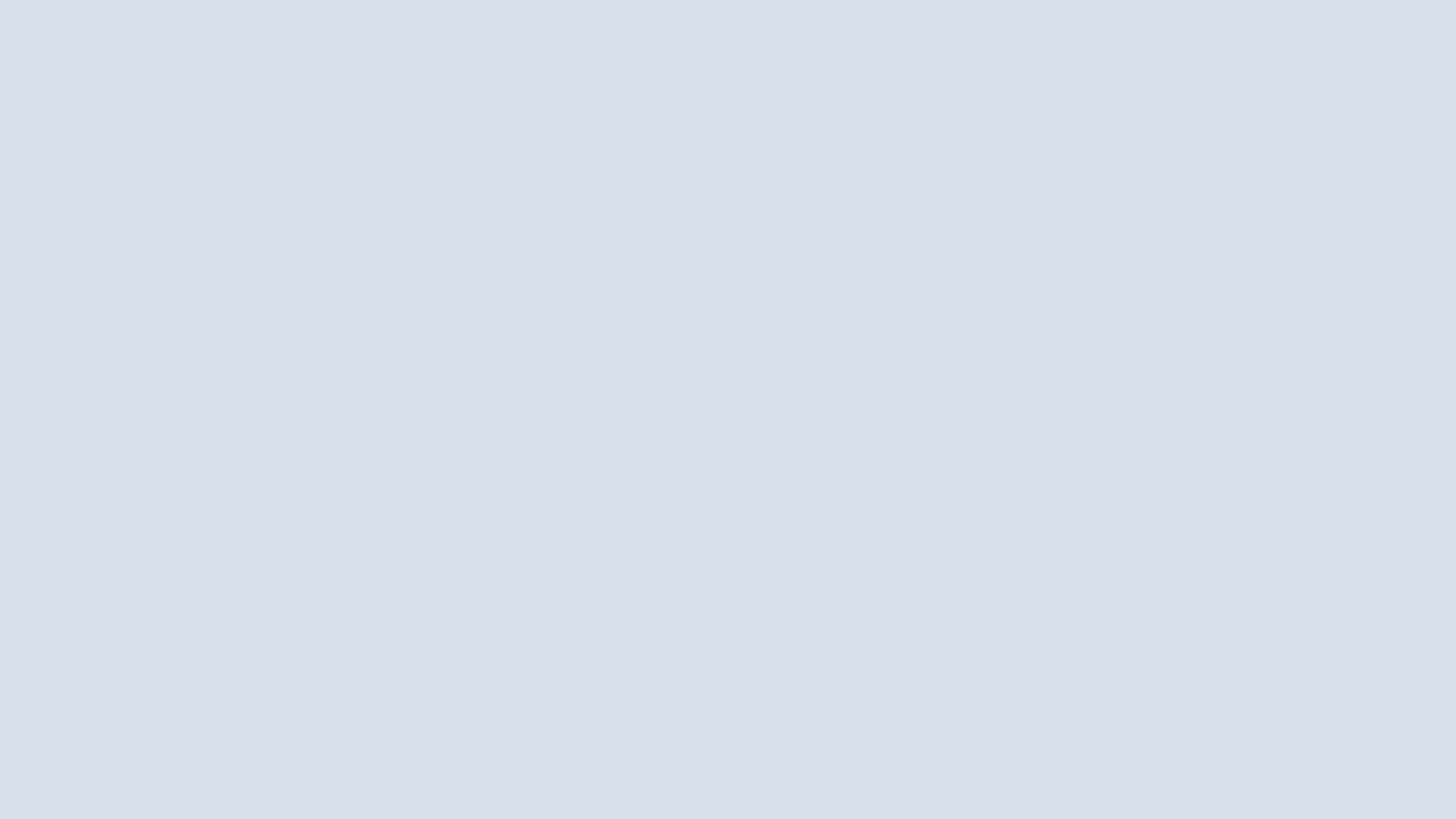The intended image did not display properly and is represented by a rectangular, grayish-blue box. The loading error has resulted in the absence of any visible content or detail in the frame.